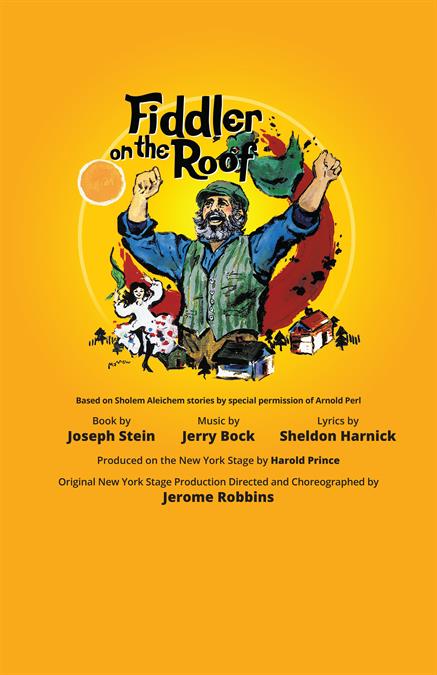The pamphlet for the musical "Fiddler on the Roof" is printed on a paper with a yellowish-orange hue resembling orange juice. At the center of the flyer is a joyful older man with outstretched arms, wearing a blue shirt with rolled-up sleeves, a greenish vest, and a green hat. His beard, a mix of black and gray, adds to his character. Behind him, a swirl of red creates a striking backdrop, where a small girl, dressed in white, is seen dancing. Below, small houses are depicted, anchoring the scene. The title "Fiddler on the Roof" is boldly written in black, with credits below: the book by Joseph Stein, music by Jerry Bock, and lyrics by Sheldon Harnick. The production was originally staged in New York by Harold Prince, with direction and choreography by Jerome Robbins.